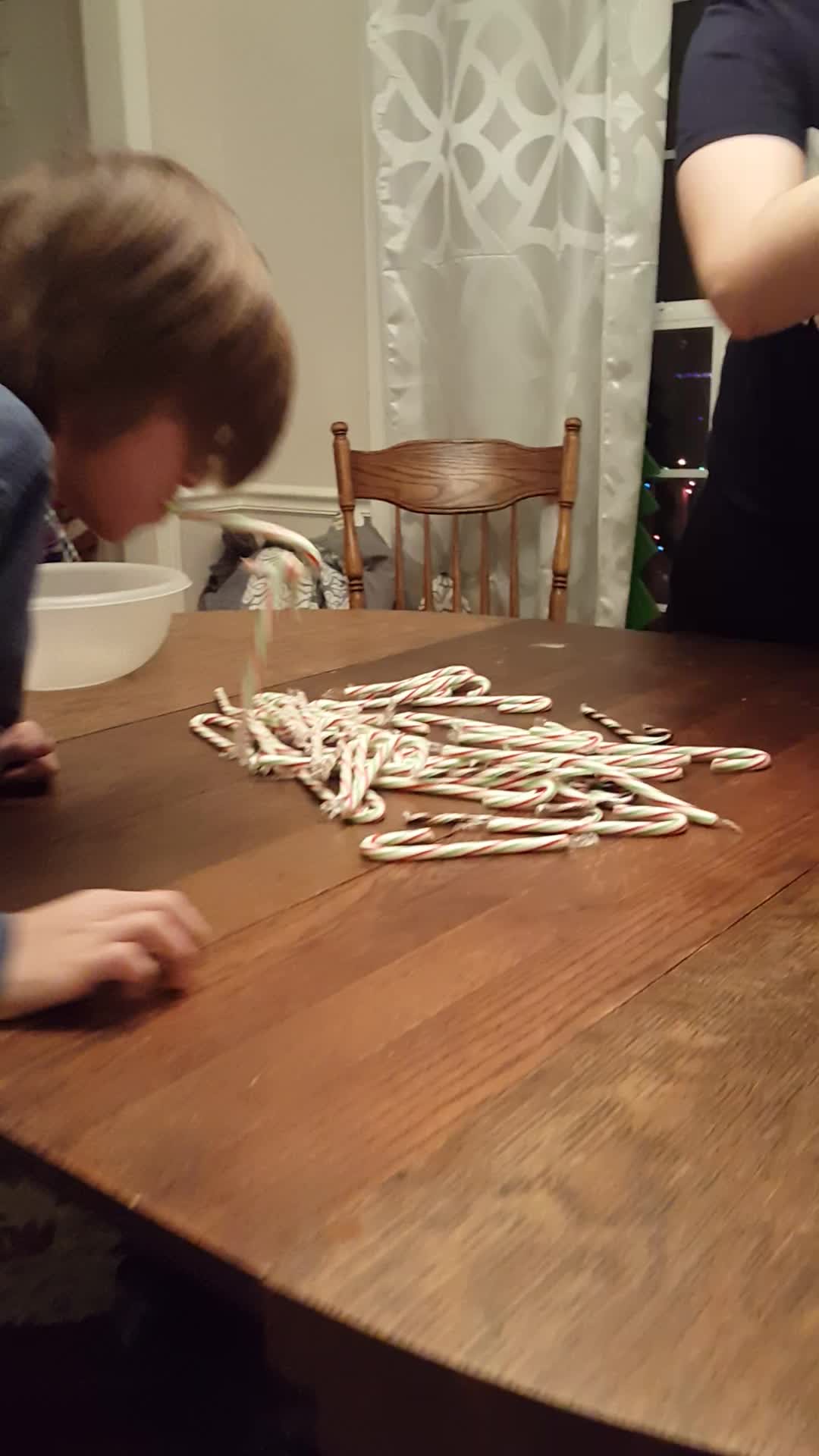This detailed color photograph captures a bustling holiday scene centered around a young boy with brown hair and long bangs, intent on a playful task at an oval-shaped wooden dining table. The table, situated in a warmly lit room with light ivory walls trimmed in white, is strewn with 20 to 30 white candy canes adorned with festive green and red stripes. The boy, with a candy cane in his mouth, uses its hook to deftly collect the other candy canes, suggesting a game akin to pickup sticks.

In the upper right corner of the image stands a woman in a short-sleeved black dress, partially visible, with her arm placed by a window dressed in elegant, silky white curtains featuring a delicate design. Below the window resides an antique wooden chair with a backrest, complementing the room's cozy decor. To the boy's left, at the edge of the table, sits an opaque plastic bowl, presumably for collecting the candy canes. Beyond the window, outside, the warmth of the holiday spirit continues with Christmas lights twinkling in the night.